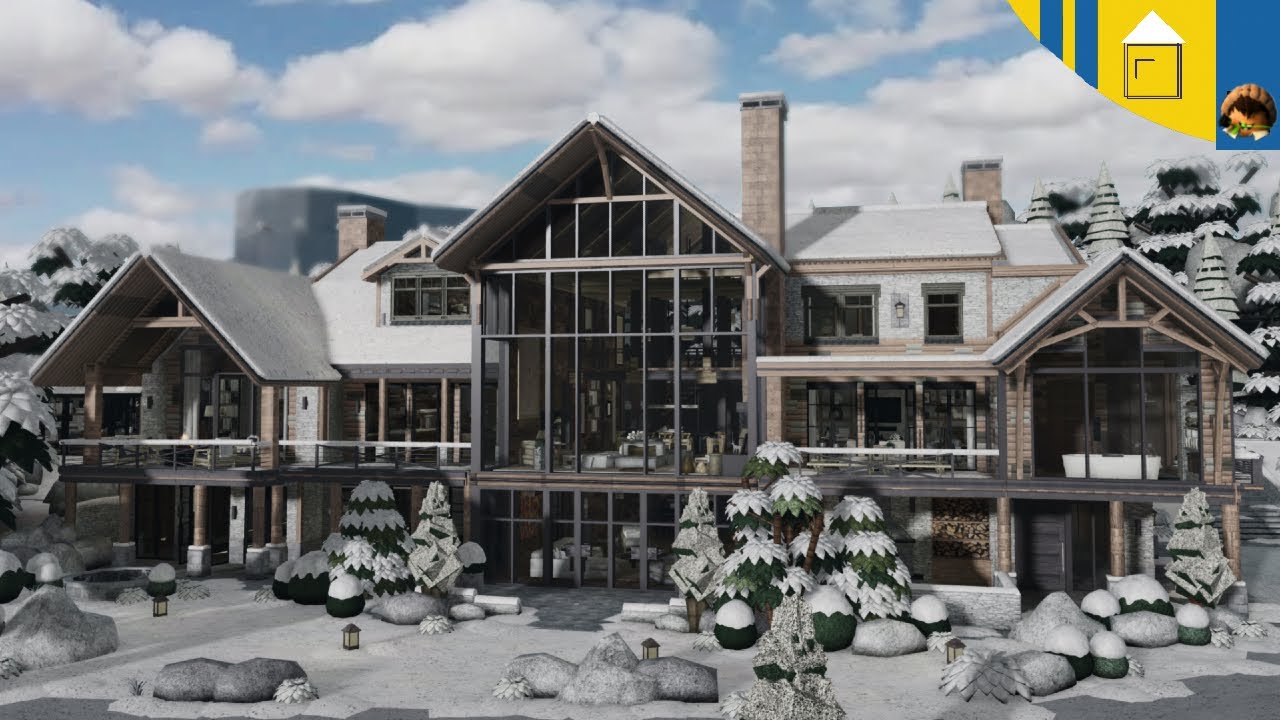The image is a computer-generated mock-up of a grand chalet-style mansion or ski lodge set in a snowy, mountainous landscape. It features a stunning front facade made almost entirely of glass, allowing a view into the interior with visible seating areas, bathtubs, and individual balconies. The building appears to have three levels, each with distinctive peaked roofs and dormers. The landscape includes snow-covered ground and artificial-looking conifers both in front and behind the structure. The scene is set on a hillside, with indications that the second level might be at ground level on one side. Additional details include several chimneys, suggesting fireplaces inside, a small pond partially visible at the edges, and a couple of decorative lanterns in the snow. The sky is a crisp blue with clouds, and there is a mysterious logo with an arc of yellow, blue stripes, and abstract shapes in the top right corner, reinforcing the sense that this might be part of a video game or architectural visualization.